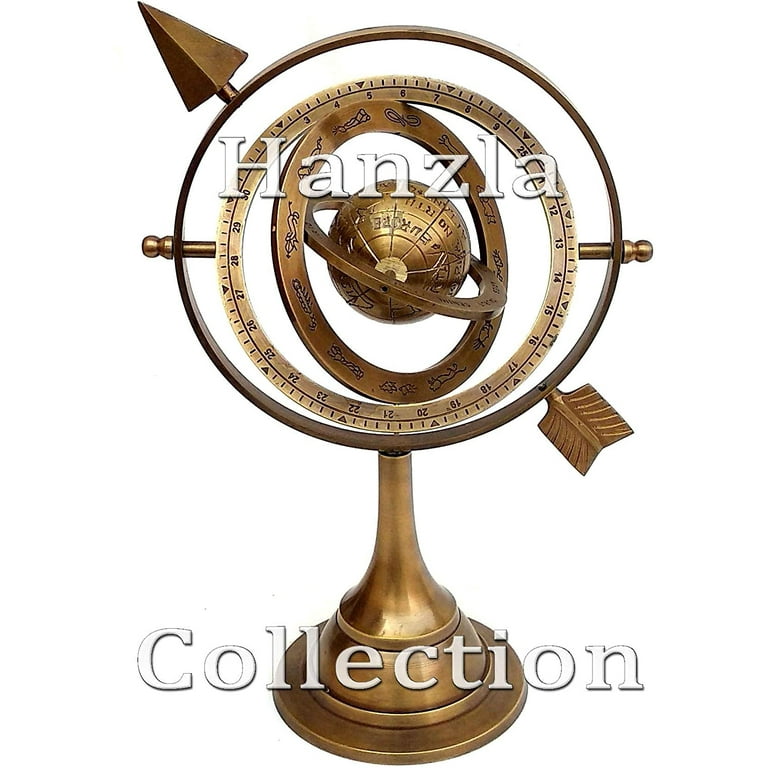In the image, there is a detailed brass object set against a pure white background. The centerpiece is a polished, golden globe that appears capable of spinning. Surrounding the globe are multiple concentric rings, each larger than the previous one, creating a complex and elegant structure. The outermost ring features an arrow, suggesting rotational movement. This design bears a striking resemblance to a large compass, complete with meticulously detailed markings and fittings that hold the concentric rings together. Adding to the intricate design, some of the rings contain constellations and ruler-like markings. The entire object culminates in an inverted, trumpet-like base. Overlaid on this sophisticated brass structure is the white text "Hansluck Collection," indicating the item's association with this collection, which might inspire viewers to explore further.